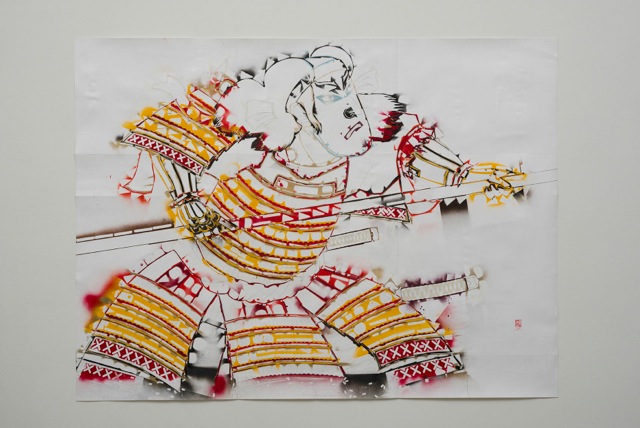This detailed artwork depicts a menacing samurai, characterized by his intense facial expression, adorned with traditional armor. The samurai's attire includes bright yellow shoulder armor with red edges marked by small white X's, and similarly patterned leg armor that transitions from yellow plates to red at the bottom. He's brandishing a cylindrical staff, held firmly in both hands, featuring red crossed marks in its central portion. His eyes are intricately outlined in blue ink, adding a touch of vividness to his stern gaze. The figure is rendered in a striking combination of black, yellow, red, and white, suggestive of watercolor or a spray paint technique. The piece is drawn on creased paper, mounted against a white background—either a wall or a tabletop. The bottom right corner of the paper features a small, indistinct red logo, further contributing to the intricate detail of the piece.